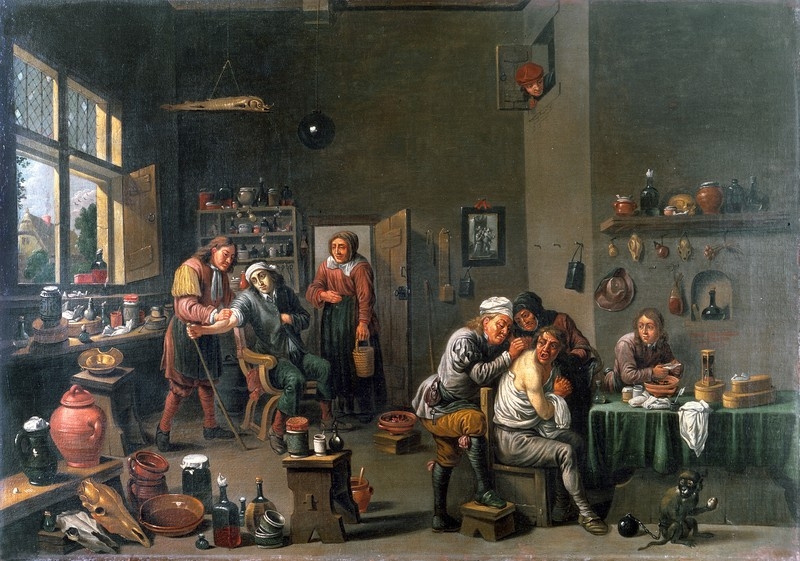The painting, an old-fashioned horizontal rectangle with no visible border, captures a detailed scene inside a grayish-brown or green room, perhaps a house, workshop, or a very old-time doctor's office. On the left, an open window with stained glass diamond patterns reveals the sky outside. Near the center left, a wooden door stands ajar, through which an older woman in a reddish blouse, long dark green skirt, and headscarf enters, carrying a pail. 

The scene is populated by several figures: one man with his shirt down sits in a chair while another stands behind him, seemingly working on his back. In the background, another man sits with a bandage around his head, extending his arm as if being tended to. Beside him, an array of small wares, including vases, bowls, and wine flasks, is scattered around a small table. To the right, a table with a green tablecloth is crowded with various medical equipment and four people: a woman handling a bowl and two men crowding around a seated man. 

In the lower right corner, a monkey further adds to the bustling complexity of the room. High above, a curious figure peeks down from a cubbyhole. The painting, likely depicting a medical scene, evokes the 1700s or 1800s through its detailed wardrobe and intricate setting.